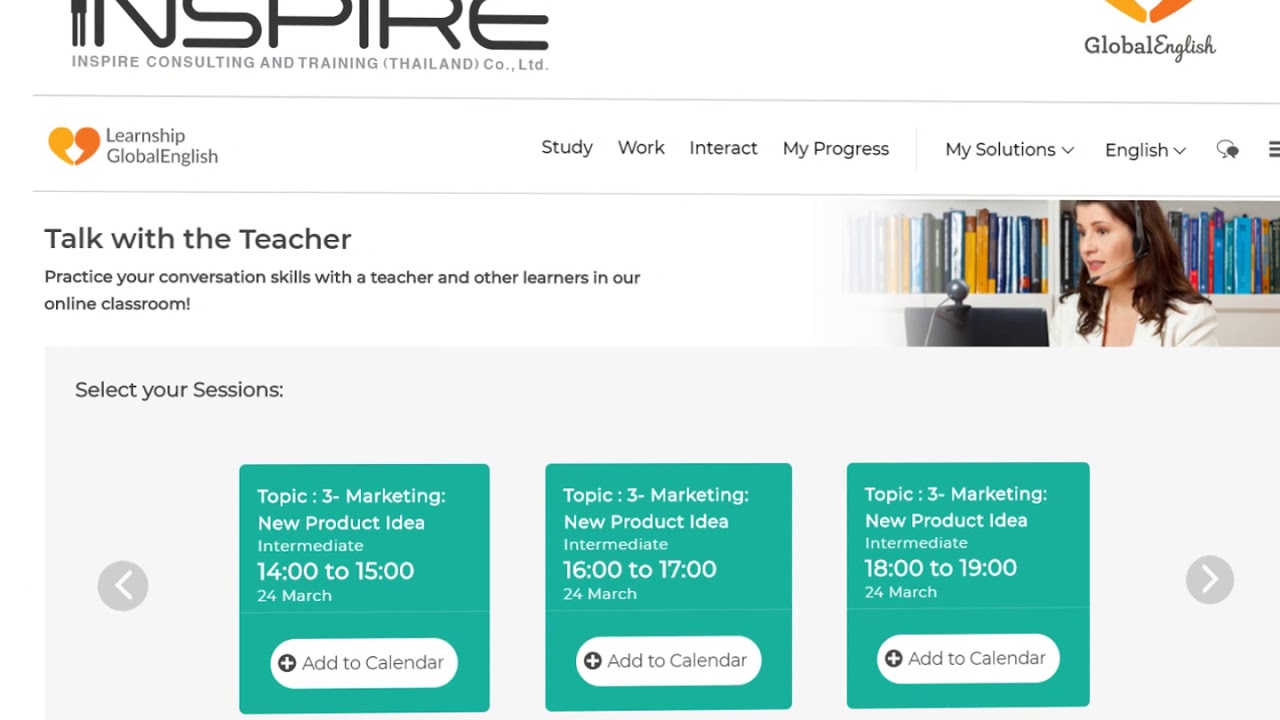---

The webpage displays a professional interface that introduces "Inspire Consulting and Training (Thailand) Co. Ltd.," though the top section, presenting the logo, is slightly cut off, leaving only half of the word "Inspire" visible in a bold black font. Beneath it, a light gray, uppercase tagline reads "INSPIRE CONSULTING AND TRAINING (THAILAND) CO. LTD." 

To the right of "Inspire," a partially obscured logo composed of light and dark orange, slanted lines forming a point, matches the incomplete top section. Underneath, the text "Global English" appears, with "Global" in print and "English" in cursive black font, separated from the next section by a faint line.

The subsequent section provides a clearer view of the full logo: a heart-like shape with the left side in light orange and the right half in brighter orange, forming two rounded loops that meet at a point at the bottom. To the right, the phrase "Leadership, Global English" is rendered, followed by menu options in a standard black font: "Study," "Work," "Interact," "My Progress," and "My Solutions" with a small down arrow by it, another "English" with a down arrow, talking bubbles, and three horizontal lines on the far right side.

Another subtle line divides this content from the next area, which is headlined with bold black text: "Talk with the teacher." Below it is the description: "Practice your conversation skills with the teacher and other learners in our online classroom!" To the right, a horizontal rectangular image shows a woman wearing a headset and a white jacket, with brown hair, looking toward the bottom left corner. She is at a computer with a bookshelf of books visible behind her.

Under this image is an off-white section starting with "Select your sessions:" followed by left and right navigation arrows. Centered are three green vertical rectangles, each detailing different session times in white font:

1. "TOPIC: 3 - Marketing: New Product Idea, Intermediate, 14:00 to 15:00, 24 March." At the bottom, a white "Add to Calendar" button with black text.

2. "TOPIC: 3 - Marketing: New Product Idea, Intermediate, 16:00 to 17:00, 24 March." Similarly, it includes a white "Add to Calendar" button with black text.

3. "TOPIC: 3 - Marketing: New Product Idea, Intermediate, 18:00 to 19:00, 24 March," also featuring the same "Add to Calendar" button.

---